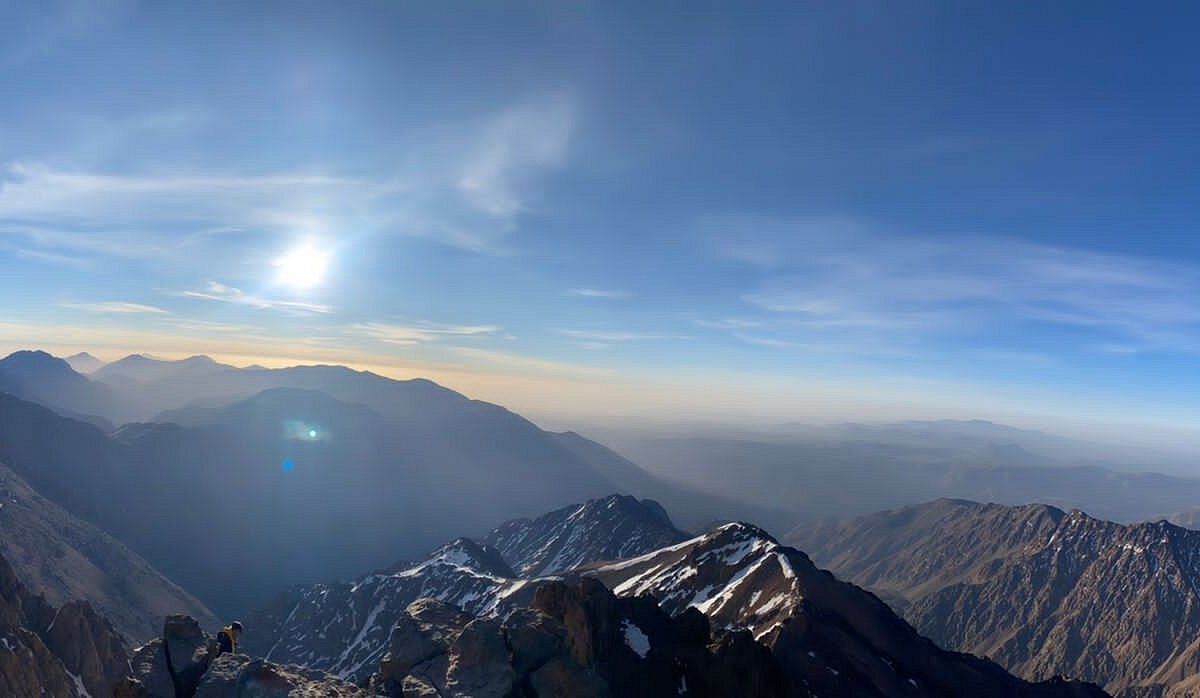This aerial photograph, taken from a high vantage point, captures a vast and rugged, unidentified mountain range. The sun is descending in the late afternoon sky towards the west, casting a yellow-golden hue over the horizon while the rest of the sky remains a deep, dark blue with wispy clouds. The foreground features a series of dark, brown, rocky mountaintops with sparse patches of lingering snow, indicating that it is not the peak of winter. The mountains stretch into the background, gradually fading into a bluish-gray haze. Near the lower left corner, a small figure can be seen, seemingly perched on the edge of a rock or boulder, dressed in a jacket with a yellow stripe down the arm and possibly a black hat or helmet. A hint of a lens flare adds a touch of realism to the shimmering sun in the upper left quadrant of the photo, which overall, appears slightly tilted with the horizon sloping downwards to the right.